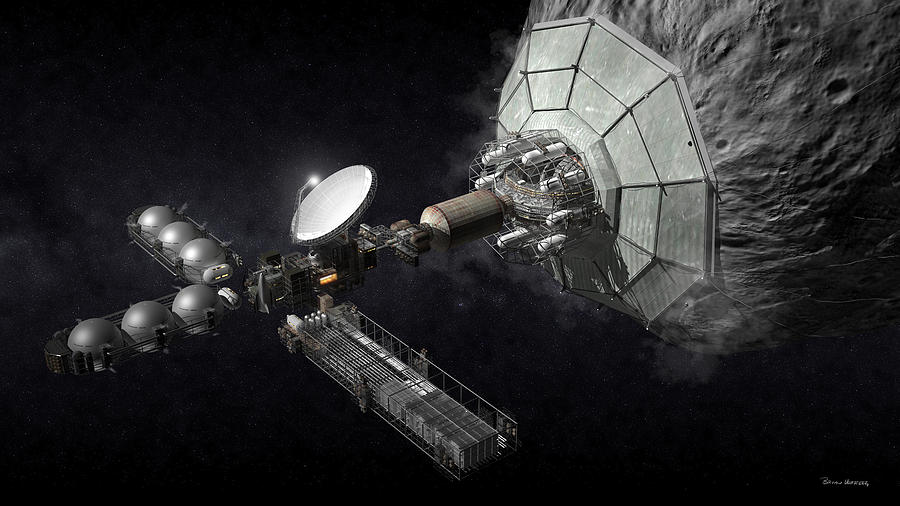This detailed digital artwork explores the futuristic concept of asteroid mining. Dominating the right side of the image is a massive gray asteroid, securely held by an intricate contraption designed for extracting valuable resources. Adjacent to this, several white tubes arranged in a circular formation are encased in a silver cage, highlighting the advanced technology involved in the process. These tubes are connected to a slightly rusted silver cylinder, which in turn links to additional sophisticated machinery composed of gleaming silver metal.

A prominent feature of the scene is a circle emitting a beam of light, illuminating the upper left part of the image and adding a sense of activity and energy. Scattered throughout the scene are several silver metal walkways, adding depth and dimension to the composition. Notably, two of these walkways, one extending straight ahead and another off to the left, each support large gray spheres, enhancing the industrial feel of this imaginative portrayal of space exploration and resource acquisition.